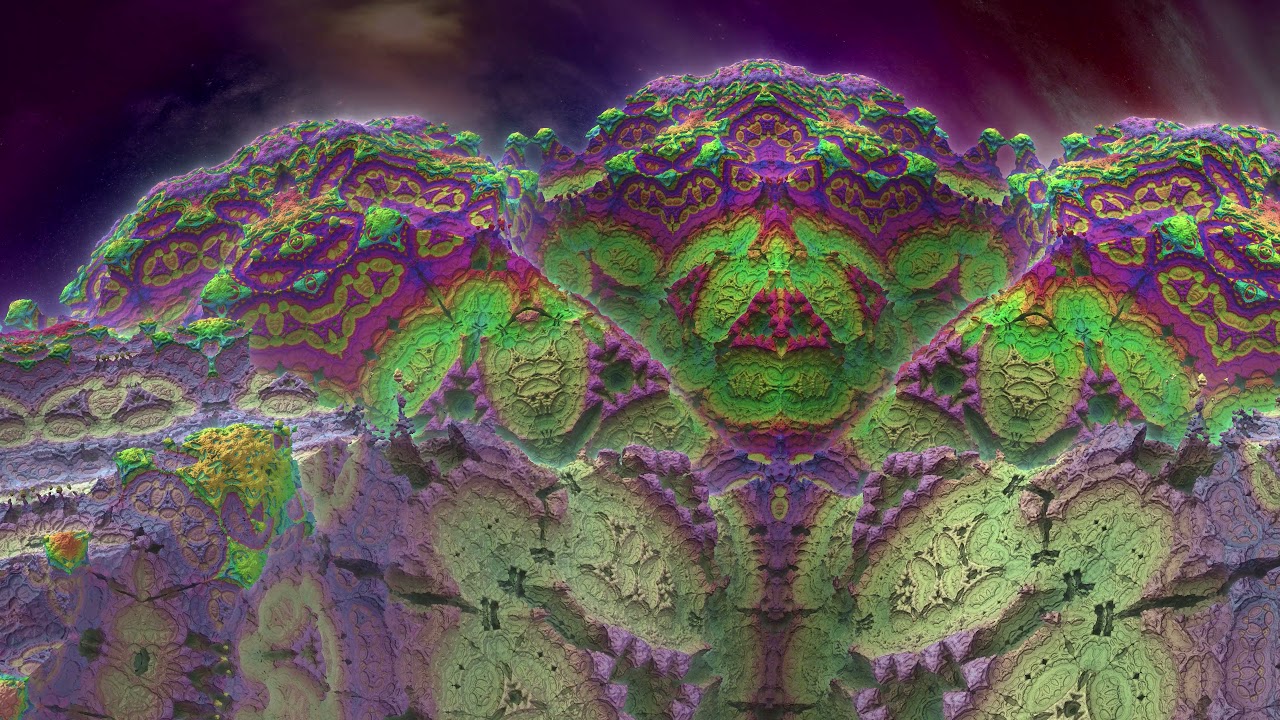The image showcases an abstract, computer-generated art piece brimming with intricate designs that recall the complexity of Paisley print. The dominant colors are vibrant and varied, with a striking bright green and brilliant purple taking center stage. Toward the top, the artwork features swirling, misty amalgamations of reds, purples, and grays, creating an ethereal atmosphere. Interspersed within the middle section are detailed images in pink set against the vivid green backdrop, including what appear to be mask-like faces or perhaps even the visage of a deity, reminiscent of Indian art.

The lower portion transitions into softer hues, with pale greens and purples that suggest a more faded appearance. Embedded within this section are forms that evoke the look of fossils or ancient fish life, lending the whole piece an almost geological feel, as if it were a painted rock formation. At this level, the designs become more indistinct, flowing into one another in a manner reminiscent of elements observed under a high-powered microscope. Overall, the topmost regions of the image are characterized by intricate, hot pink and purple patterns that appear to emanate light against an enveloping dark purple background. The cumulative effect is a strikingly detailed and mesmerizing interplay of colors and forms.